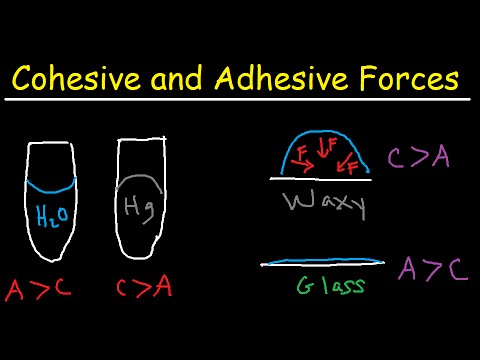The image is a simple infographic with a black background, created with basic digital tools, possibly something like Windows Paint. At the top, in yellow letters with a white underline, it reads "Cohesive and Adhesive Forces." On the left side, there are two white, flat-topped pill shapes. The first pill shape, labeled "H2O" in blue, has "A > C" written in red beneath it. The second pill shape is labeled "HG" in gray, with "C > A" written in red below it. On the right side, there's a blue dome with a white line, labeled "waxy" with the text "C > A" in purple beside it, and red arrows pointing towards the center. Below this, there's a depiction resembling a side view of a plate or a flat surface, indicated by a white line and a small teal line, labeled "glass" in green, with "A > C" written in purple to the right. The infographic appears like a snapshot from an educational video, illustrating the concepts of cohesive and adhesive forces.